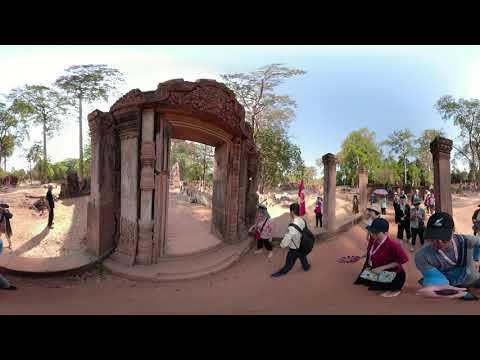This photograph captures a detailed and vibrant outdoor scene at what appears to be an ancient stone temple under a bright blue sky. The temple's focal point is a large, intricately carved square entryway made of a soft brownish clay-like material. Surrounding the entryway are several decorative, square-shaped stone pillars. A mix of curious tourists, many equipped with dark baseball caps and various backpacks, are scattered around the scene; some are walking towards the temple, others have already passed through the entryway. In the background, tall trees with bright green leaves frame the temple, adding to the lively atmosphere. The ground is a light beige-brown, contributing to the overall earthy feel of the photograph. One notable individual in the foreground, possibly the photographer, is a man with short black hair, wearing a black hat and a blue long-sleeve shirt. The image is enclosed by long vertical black bars at the top and bottom, accentuating its panoramic view. Despite some variations in activity, the overall scene is dynamic, capturing a moment of exploration and historical appreciation on a sunny day.